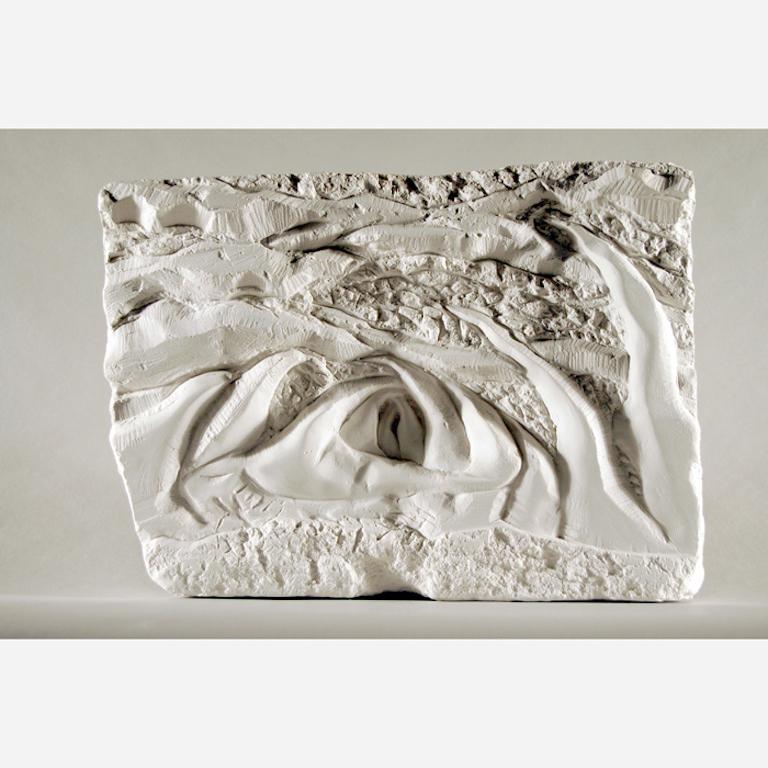This photograph captures a roughly square-shaped stone carving, set against a white background on a white counter, creating a stark, all-white backdrop. The carving itself appears to be made of marble or sandstone, characterized by an intricate interplay of intersecting lines and jagged edges, giving it an uneven, hand-chiseled appearance. Central to the piece is a prominent, cave-like divot or hollow that some might interpret as resembling an eye, adding an enigmatic focal point to the artwork. The carving features a variety of textured grooves and wave-like patterns that evoke natural erosion processes, whether by wind or water, adding to its organic aesthetic. The square slab is not perfectly uniform, suggesting it has been manually shaped or carved, with a blend of thick and skinny lines creating a complex, almost cavernous landscape on its surface.